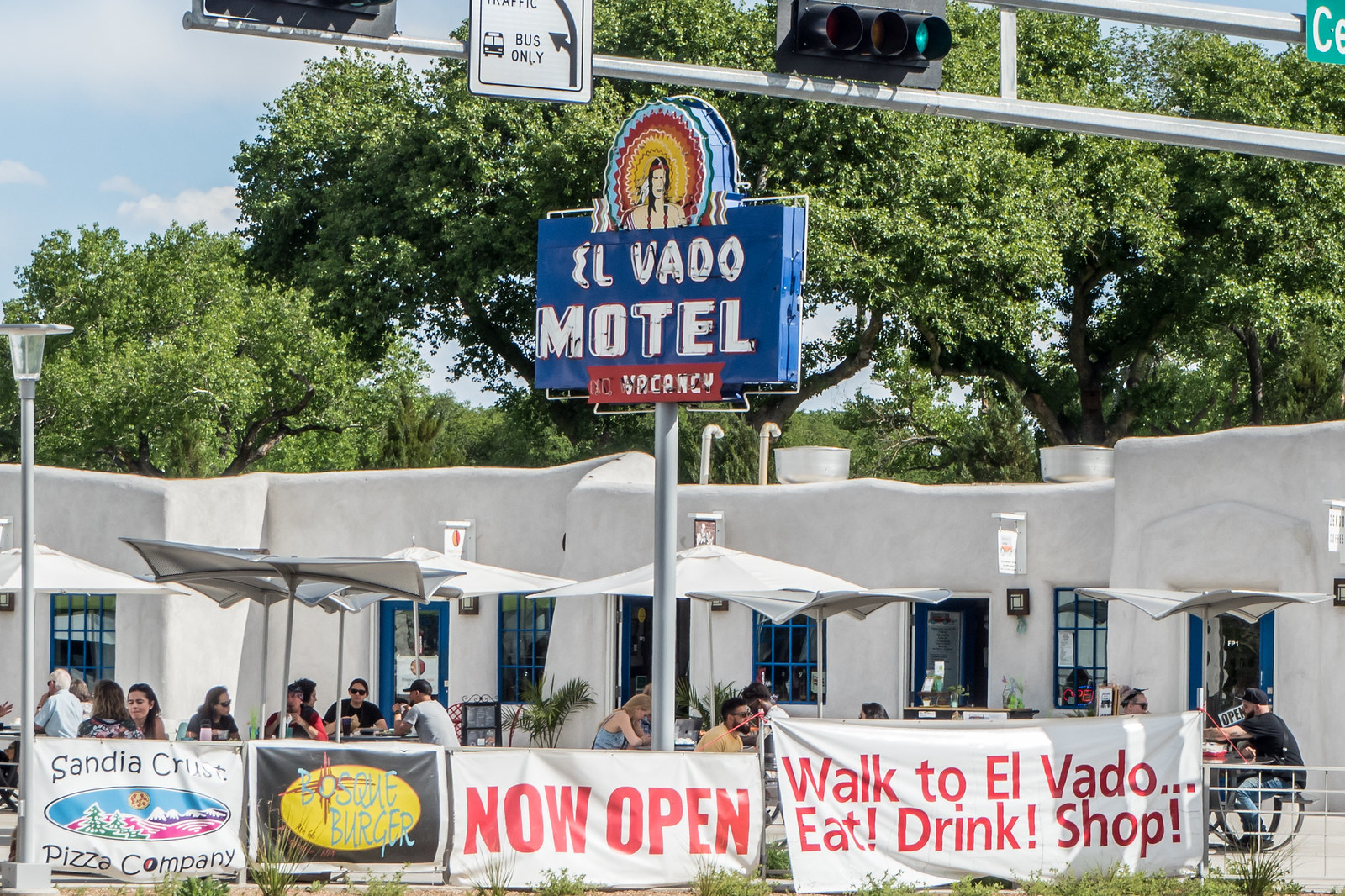This outdoor photograph captures the El Vado Motel, a horizontal one-story white stucco building featuring many windows with blue frames, aligned in a southwestern Pueblo-style design. The scene includes a vibrant patio area in the foreground, furnished with tables and white market-style umbrellas under which people are dining. Central to the image is a prominent sign elevated on a tall silver pole. The sign features a blue background with white text that reads "El Vado Motel," and below it, a red rectangle with white lettering indicating "Vacancy." At the top of the sign, an illustration shows a Native American figure within a circle framed by a red and yellow sunburst.

In the background, large green trees with dense foliage are set against a blue sky dotted with white clouds. Along the bottom of the image, a row of horizontal banners advertises various businesses: "Sandia Crust Pizza Company," "Bosco Burger," a "Now Open" announcement, and "Walk to El Vado... Eat! Drink! Shop!" The scene merges the charm of southwestern architecture with the lively ambiance of an outdoor dining area.